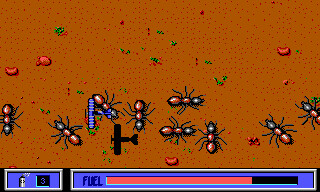The image depicts a vintage video or computer game, likely from the late 1990s or early 2000s, featuring a dirt landscape dotted with small rocks and patches of greenery. Toward the bottom of the screen, ten ants are scattered around, seemingly engaged in a puzzle-like activity where they pick up and place objects. The interface indicates that one of the ants is nearly at full fuel and has approximately three lives remaining. The graphics are relatively simple, characteristic of older computer games, enhancing the nostalgic feel of the scene.